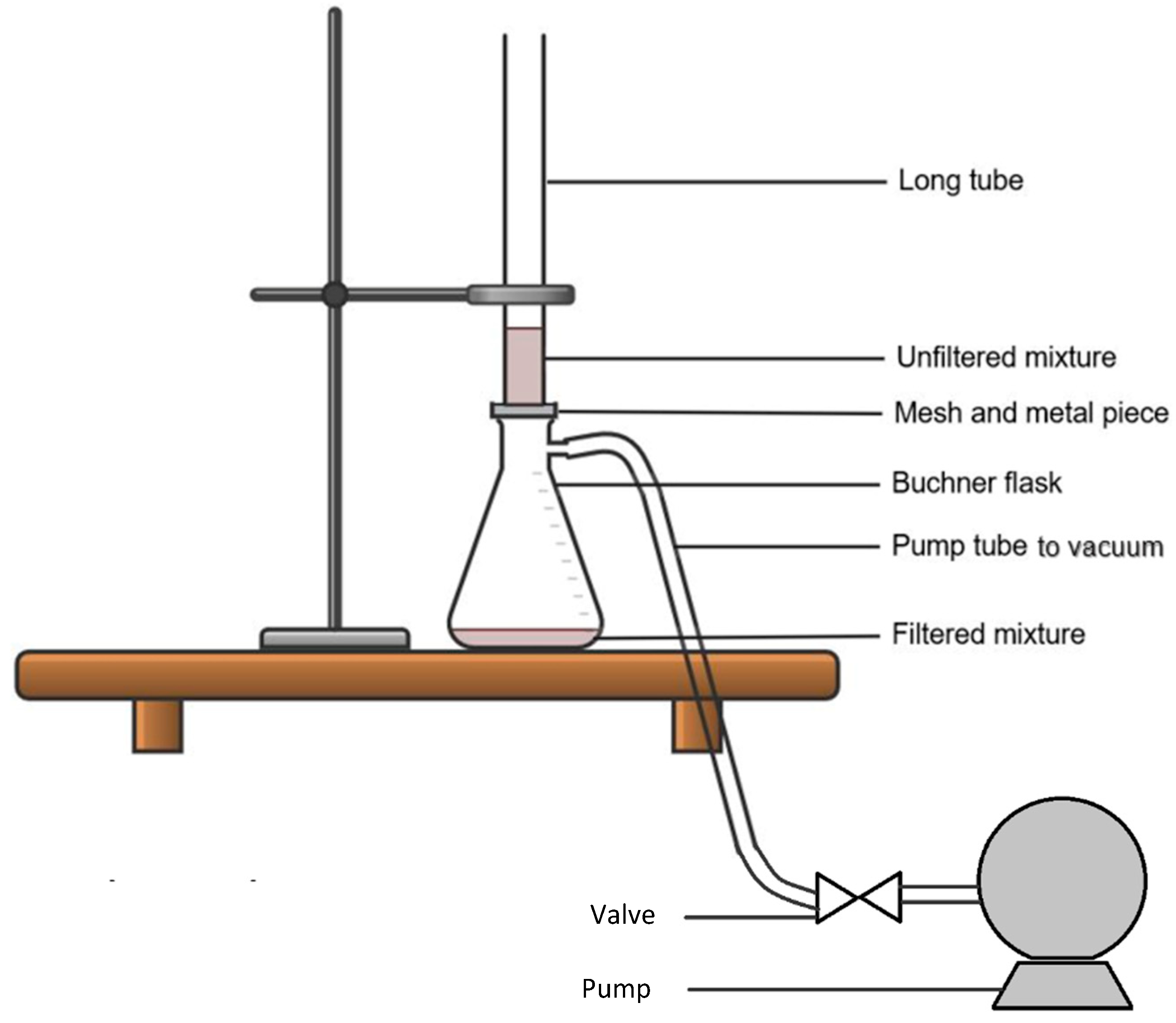The image is an animated illustration of a chemistry experiment set up on a horizontal wooden shelf with small legs. At the center of the illustration sits a Buechner flask, containing a bit of filtered pink liquid at its bottom. A long tube extends vertically out of this flask, held up by a silver or gray ring stand on the left. This long tube, labeled 'Long Tube,' leads to a mesh and metal piece at the opening of the flask, capturing the unfiltered mixture. From the flask's side, another tube extends to the right, leading to a gray valve and a gray trapezoidal pump labeled 'Pump,' indicating it's part of a vacuum system. The text in the image provides labels and explanations for each part of the setup, including 'Unfiltered Mixture,' 'Filtered Mixture,' 'Mesh and Metal Piece,' and 'Pump Tube to Vacuum,' making the scientific process easy to understand. The background is completely white, emphasizing the simplicity and educational purpose of the illustration.